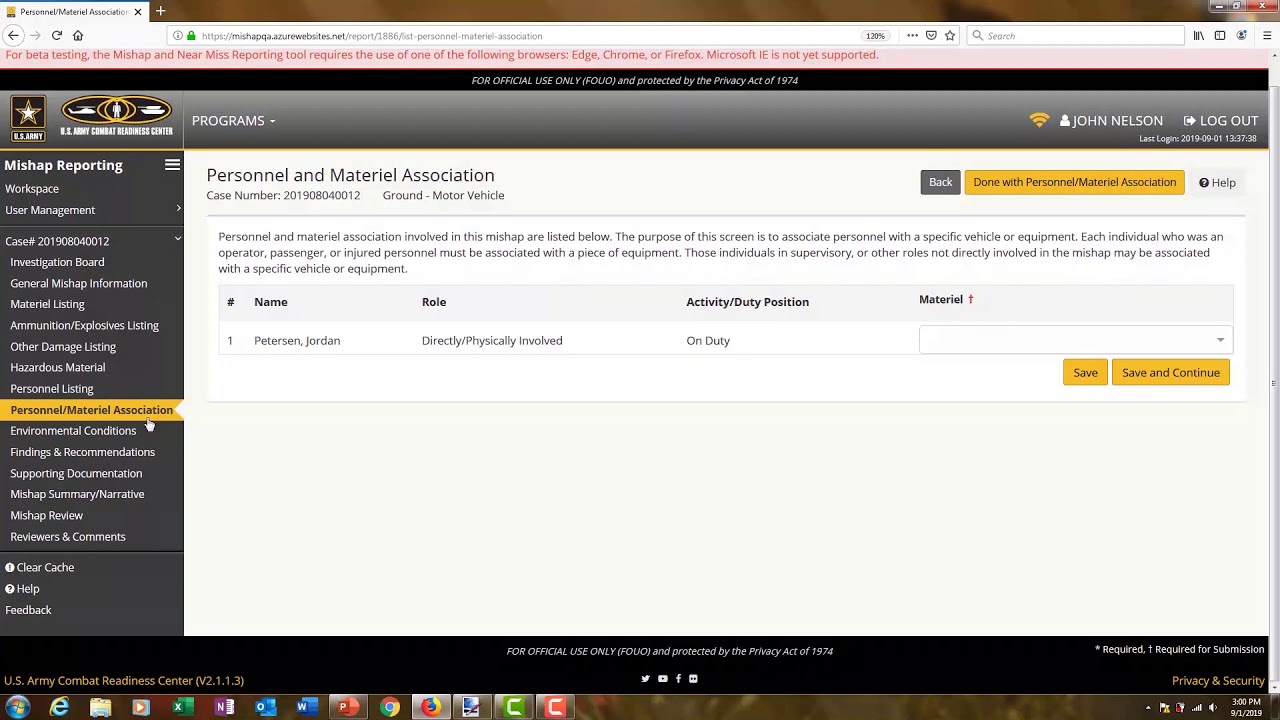**Detailed Caption:**

This image is a screenshot from a Windows Vista operating system, displaying a webpage used for the US Army's mishap and near-miss reporting tool. At the top of the screenshot, there's a gray bar with black text stating "Personalized Material and Association," accompanied by a black "X," a purple and white plus sign, and a black and white circular icon. On the right-hand side of this bar, there are the typical window control icons for minimize, resize, and close, also in black.

Directly below, the content section has a gray background with text explaining that the tool is intended for beta testing and recommends using Edge, Chrome, or Firefox browsers, while noting that Microsoft Internet Explorer is not supported. The US Army logo is present, indicating the affiliation.

On the right side, there's the name "John Nelson" alongside a prominent "Logout" button. Below this, in a black background with white text, various sections of the tool are listed: mishap reporting workspace, user management, cache, investigation board, general mishap, among others. The small text in this section is partially illegible due to its size.

Following this, the main content area is on a white background with black text displaying "Personnel and Management Association," a specific case number, and details about a ground vehicle motor incident. The interface includes buttons for navigation—a "Back" button, "Save" and "Discard" options, as well as sections detailing the personnel involved in the incident and their duty status at the time.

At the bottom of the screenshot, the Windows taskbar shows, with the system time indicated as 3:00 PM on September 1, 2019.

The accompanying text also includes a heartfelt thank you and farewell message from Matt, expressing appreciation for participation in a series of unspecified activities that took place from late April to early May, and resumed in June through the beginning of July.